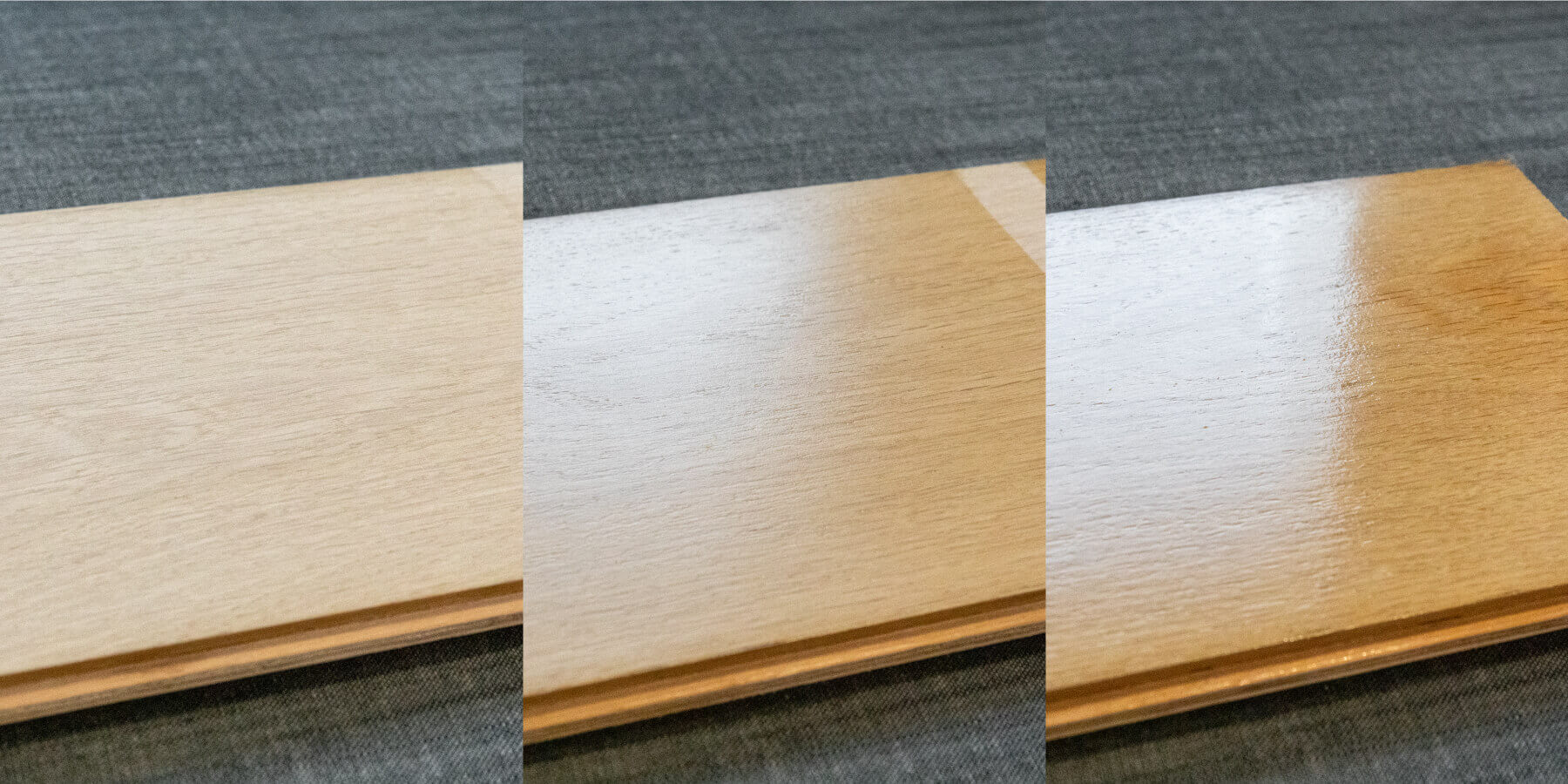The image is a detailed triptych showcasing the transformation of a light brown wooden board with a glossy finish, set against a dark gray, corporate-style carpet backdrop. Each of the three equal-sized rectangular photos, arranged horizontally, depicts a different stage of applying the finish. In the first image, the wooden board appears unfinished, lacking any sheen or coating. The middle photo displays the board midway through the finishing process, with a partial shiny coating. The third and final image reveals the board with a complete, glossy finish that reflects sunlight from a nearby window. The meticulous progression highlights the wood's transformation, emphasizing the differences in texture and sheen throughout the finishing stages.